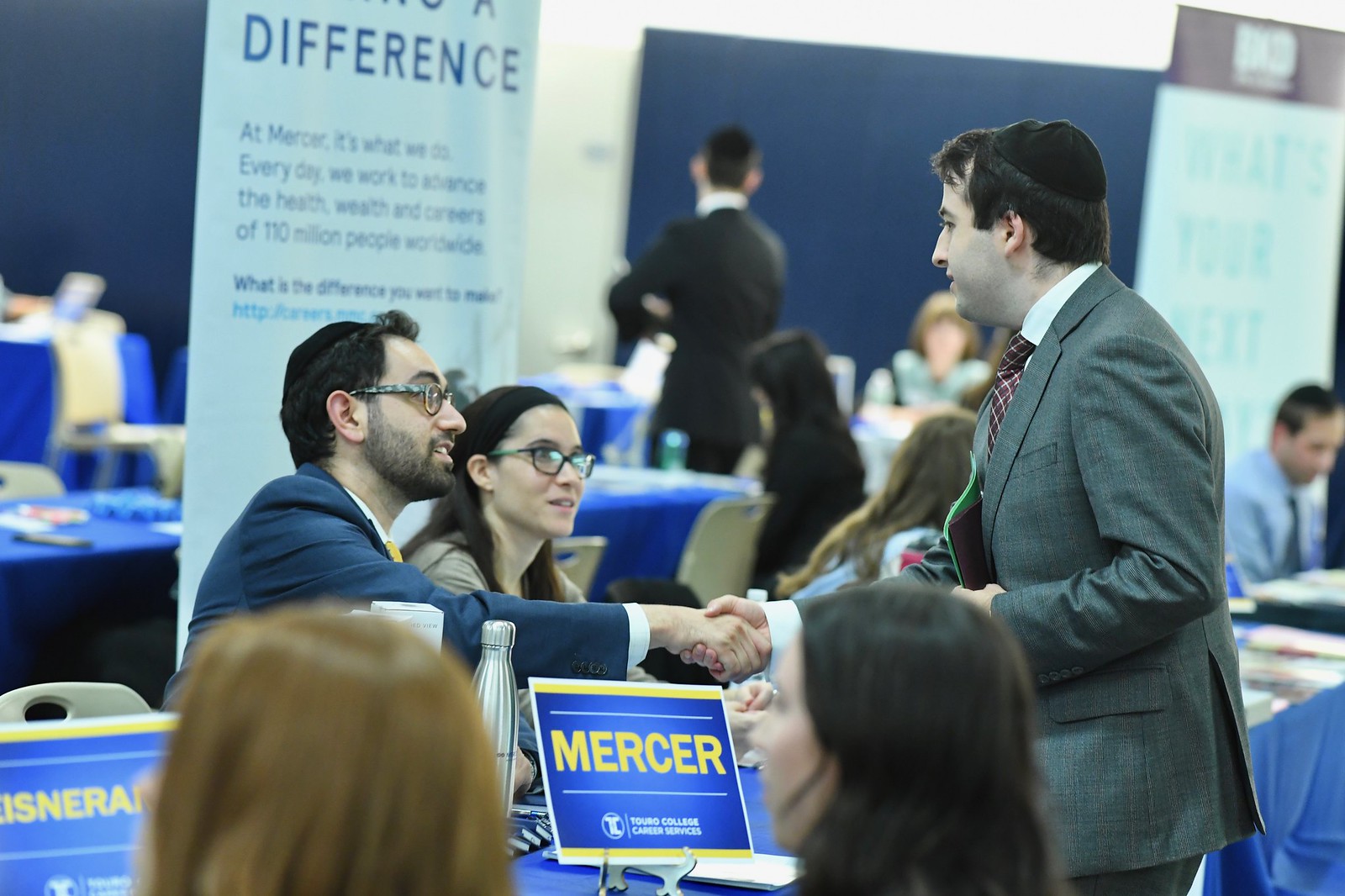This photograph depicts a career services event, likely a college or job fair, held indoors with multiple tables lined up. Each table is draped with a blue tablecloth, and focal to the image is a table featuring a sign labeled "Mercer Touro College Career Services." At this table, a man in a gray suit with a maroon tie, white collared shirt, and black yarmulke is standing and shaking hands with another man seated across the table. The seated man, wearing a blue suit, yellow tie, white collared shirt, glasses, and a yarmulke, is joined at the table by a woman with long brown hair and glasses. The table is also adorned with a silver water bottle and several pens laid out on papers. Additional signage behind them reads, "At Mercer, it's what we do every day. We work to advance the health and wealth and careers of 110 million people worldwide." Around them, several other attendees can be seen sitting at their respective tables, but the focus remains on the handshake symbolizing professional networking in progress.